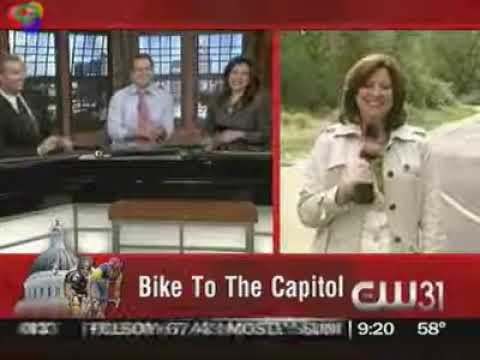The image appears to be an older screenshot from a CW31 morning newscast, which prominently features a banner at the bottom that reads “BIKE to the CAPITOL” in white font on a red background. Above this banner, a superimposed image shows two cyclists riding their bikes with the Capitol building, featuring a right circular body and dome-shaped grey top, in the background. Just below this eye-catching graphic, another black banner displays the time as "9:20" and the temperature as "58 degrees Fahrenheit," although the AM or PM distinction is not specified due to the blurred text in the screenshot.

The newscast includes two separate images: on the left, three news anchors—two men and one woman—are seated at a black desk, smiling and laughing as they report. Behind them, the windows reveal the city skyline. On the right side of the screen, a female field reporter, smiling and holding a microphone in her right hand, stands in front of a road, seemingly reporting live. She is dressed in a white trench coat, suggesting it is sunny yet possibly crisp outside, as indicated by the temperature on the screen.